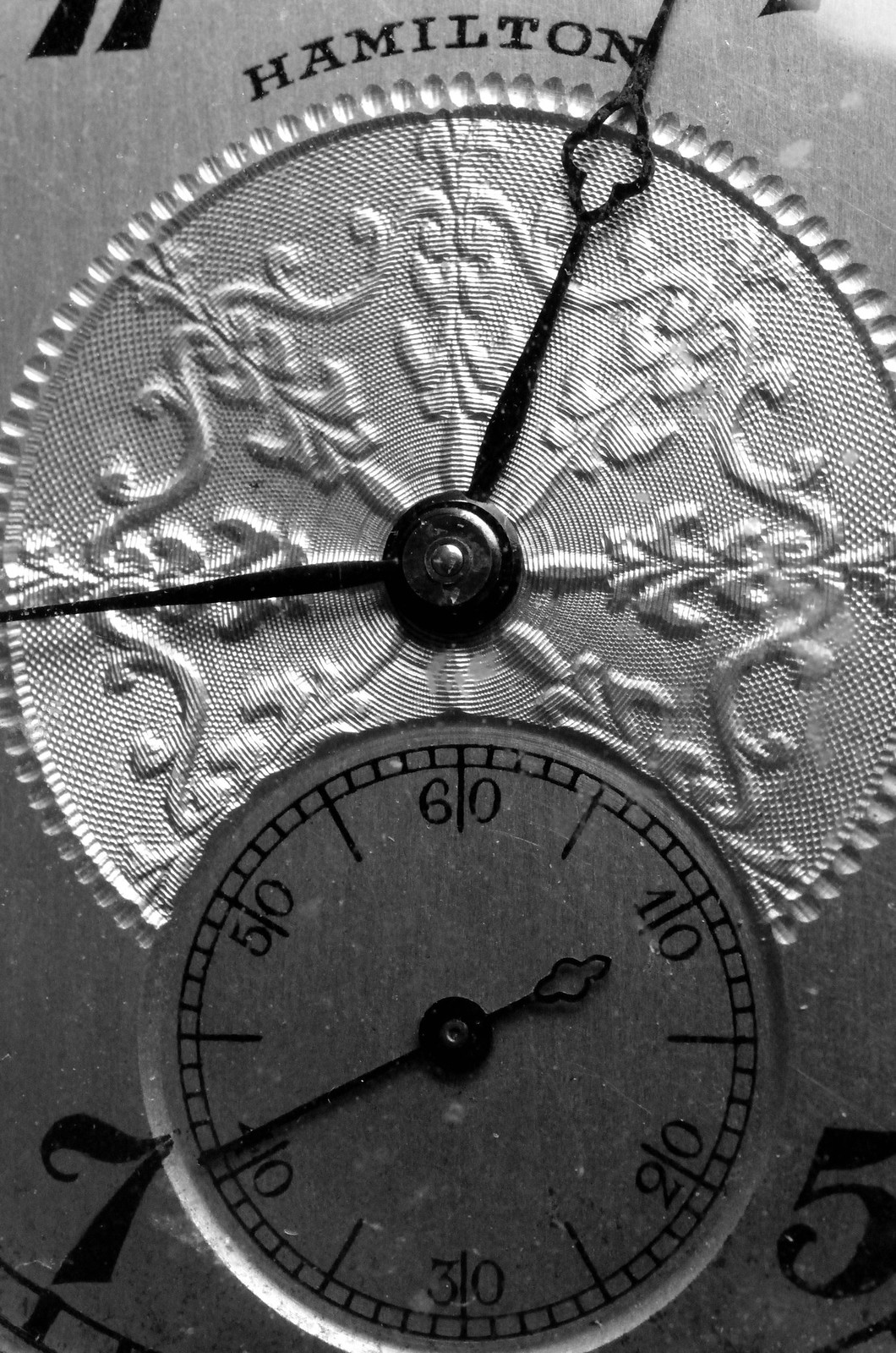This black and white close-up photograph captures an intricate detail of a Hamilton clock's face. The image is so magnified that the primary clock face is not visible; instead, it focuses on specific components. Prominently displayed is the name "Hamilton," denoting the clock's manufacturer. Below the Hamilton branding, a circular silver design is embossed on the metallic surface of the clock face. This design features a finely patterned texture, reminiscent of a floor design, and includes two small hands, possibly indicating a secondary function or measurement. Beneath this design lies a smaller circle marked with numbers ranging from 10 to 60. These numbers suggest the presence of a temperature gauge, adding to the clock's functionality. The meticulous craftsmanship and subtle features highlighted in this image convey the elegance and precision of the Hamilton clock.